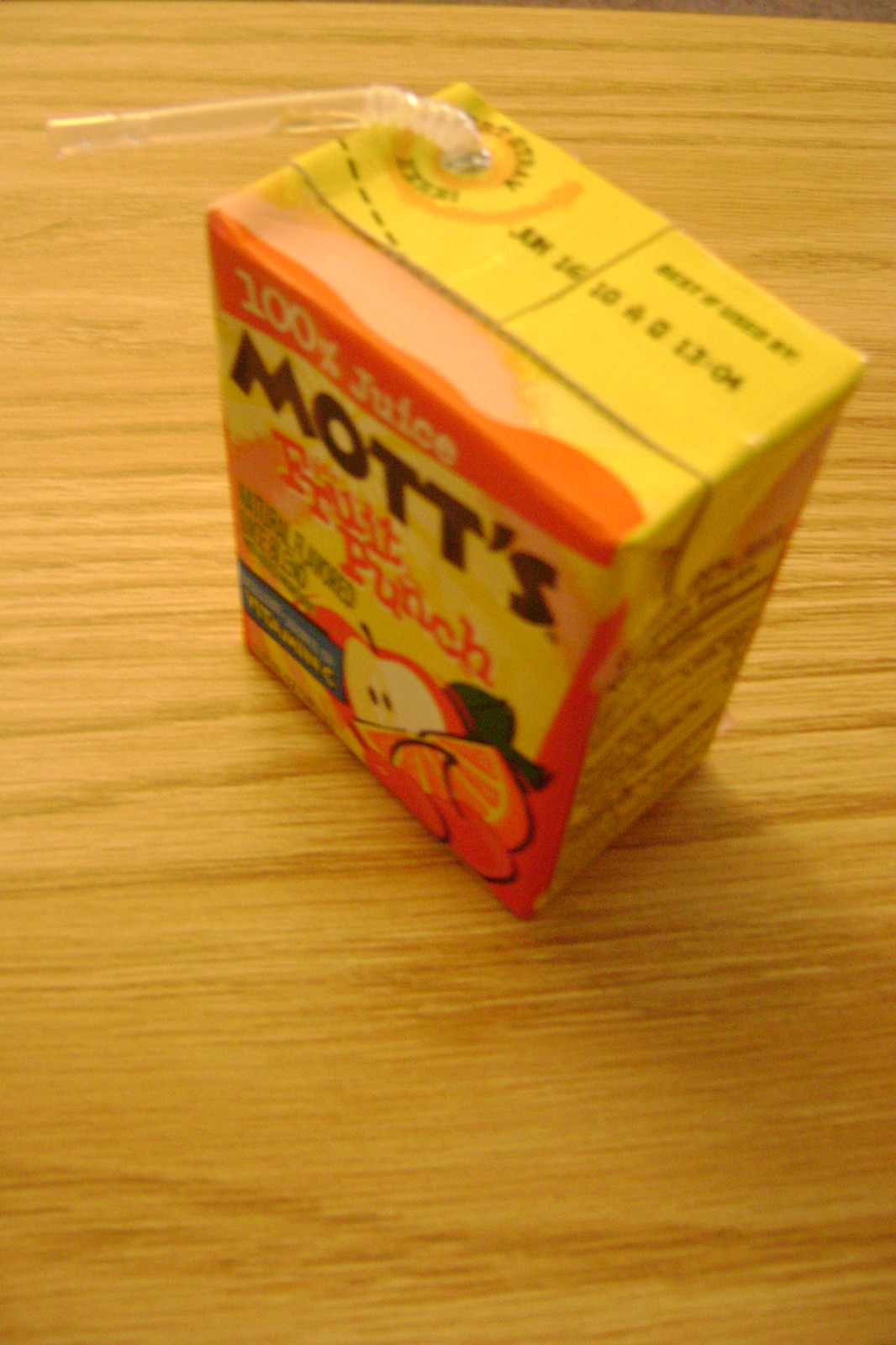This is a detailed photograph featuring a box of Mott's 100% Juice Fruit Punch, commonly enjoyed by children. The box is placed on a wooden or laminate countertop, which has a light gold hue with horizontal wood grain patterns. The photograph is taken from a top-down perspective, clearly showing the drink box with a straw already inserted and bent forward. 

The back of the juice box is yellow, while the front top portion has a pink background with bold text. The text displays "100% Juice" prominently at the top, followed by the brand name "Mott's" and then the flavor "Fruit Punch" below it. The lower right of the front face features a vibrant illustration showcasing a sliced apple along with hints of orange and possibly other fruits, incorporating a mix of orange, red, and green colors that add to the box's appeal.

At the top of the box, although blurry and unreadable, there likely is an expiration date. The overall composition of the image highlights the colorful packaging of the juice box against the subtly patterned counter, capturing the essence of a commonly seen scene.